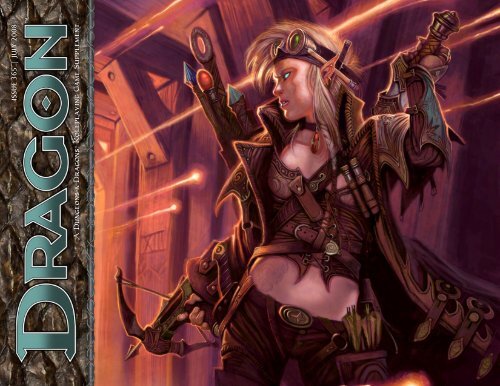This image, likely a cover from a video game or a computer-generated illustration, features an anime-style female character who appears elven with distinct pointy ears. She stands prominently to the right, drawing attention with her serious, glowering expression and cyberpunk-inspired aesthetics. Her attire includes a revealing brown leather ensemble adorned with medieval golden emblems and buckles, a headband with a green jewel, and a pair of green-lensed goggles resting on her forehead. She holds a crossbow in her right hand, armed with green-feathered arrows, and her left hand grips a sword ready for action, with more swords visible strapped to her back and one side.

The scene is dynamic, with streams of orange light or laser beams shooting horizontally across the image, creating a sense of movement and intensity. The beams culminate in bright yellow flares upon impact. The background resembles a wooden tavern, characterized by dark wooden posts and a ceiling, enhancing the medieval atmosphere. On the left side of the image, text vertically spells out "Dragon" in blue, accompanied by additional white text that is blurred and illegible. A border resembling dark gray dragon scales frames the image, tying together the fantasy elements.